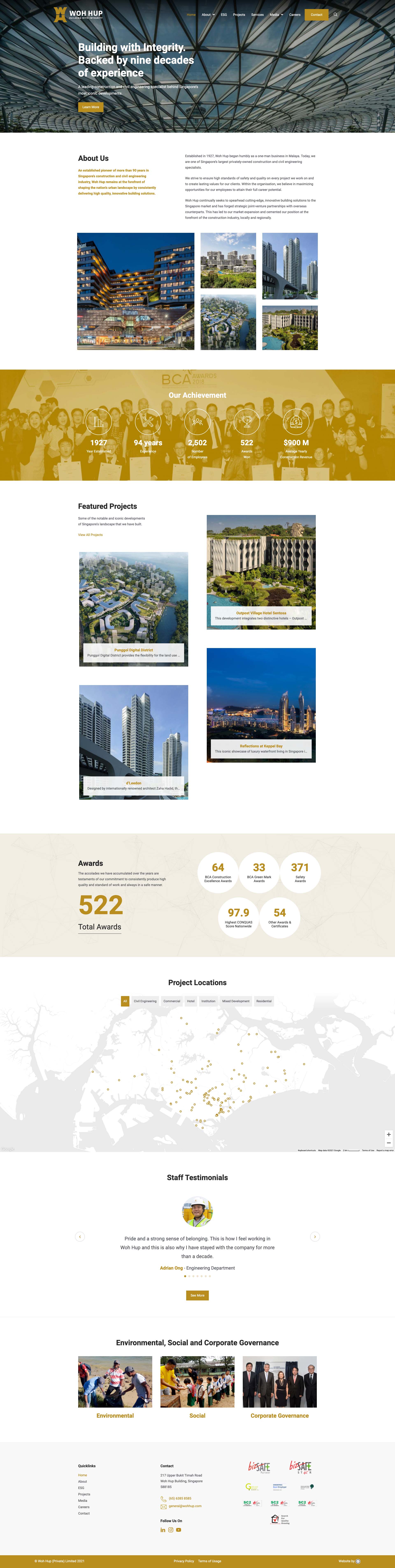A long webpage has been condensed into an image, making it difficult to read. At the top, a banner proudly states "Building with Integrity, Backed by Nine Decades of Experience," suggesting the image is from an architectural firm's website. The visible portion features a sophisticated, modern ceiling design with skylights and trellis-like elements. Although much of the text is unreadable, the image is populated with various pictures and blocks of text, primarily showcasing standard architectural projects such as hotels and office buildings. A number, "522," which might refer to awards, is also visible. Additionally, there's a map that likely indicates the locations of their projects, but the details are unclear. Scrolling further down, the image includes sections for testimonials and contact information. The background is predominantly white, with accents of yellow and light gray. A prominent image near the bottom displays a large portion of the firm's staff.